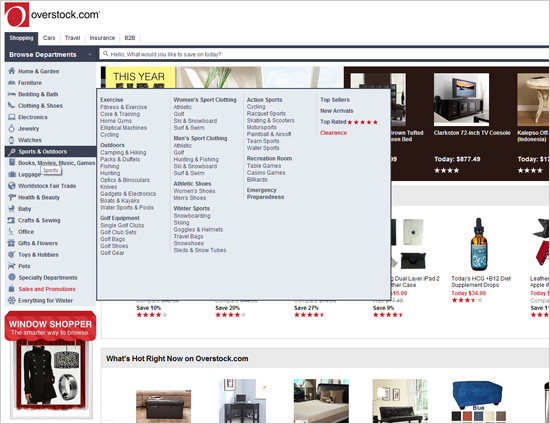The image is a screenshot from the Overstock.com website. In the upper left corner, there's a prominent square red box featuring a white "O" inside it. To the right of the box, the bold black text "Overstock.com" is displayed. Below, a navigation bar lists various tabs: Shopping, Cars, Travel, Insurance, and B2B. The "Shopping" tab is currently selected, shown with white text against a black background.

The left sidebar displays a vertical menu under the header "Browse Departments," listing various categories. The categories in order are: Home & Garden, Furniture, Bedding & Bath, Clothing & Shoes, Electronics, Jewelry, Watches, with "Sports & Outdoors" being highlighted in black, indicating it's the selected category. The list continues with Books, Movies, Music, Luggage, World Stock Fair Trade, Health & Beauty, Baby, Crafts & Sewing, Office, Gifts & Flowers, Toys & Hobbies, Pets, Specialty Departments, and Sales & Promotions (in red text). At the bottom of the sidebar, there’s a seasonal promotion titled "Everything for Winter."